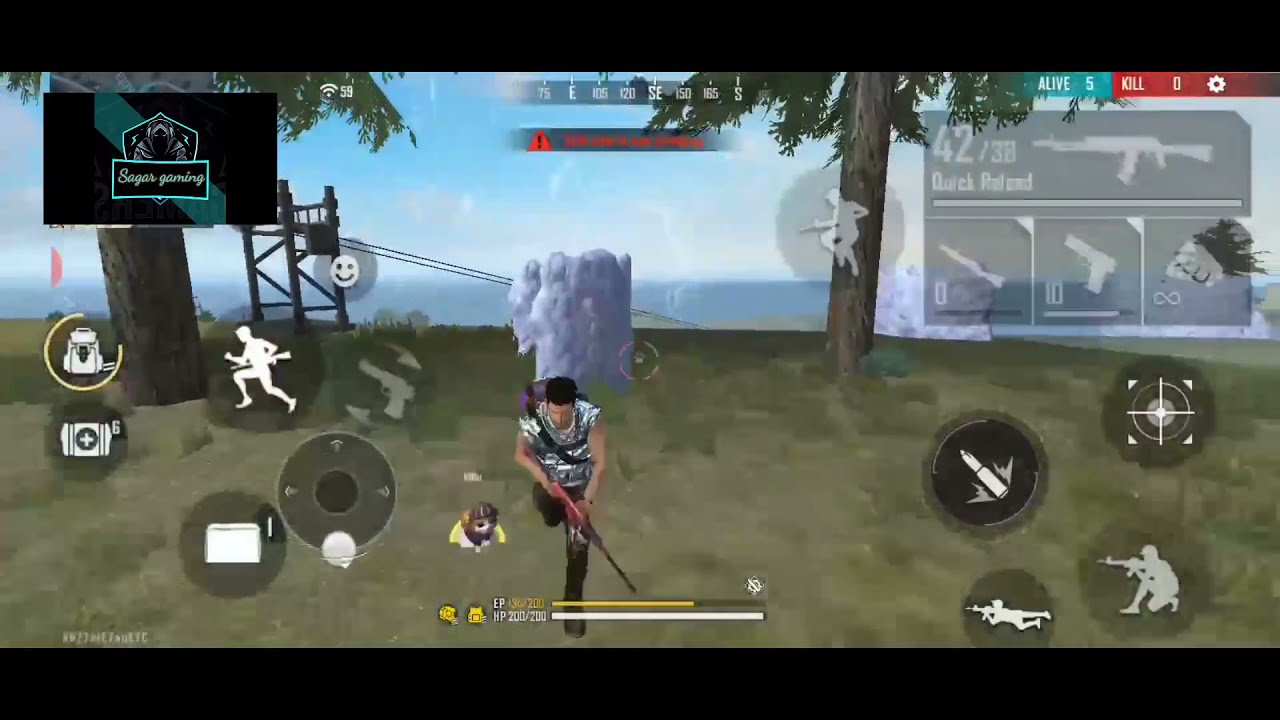The image depicts a video game screen, likely from a mobile shooter game. Dominating the foreground is a character in a short-sleeved tank top with straps, dark pants, and a backpack. He has dark hair and holds a rifle as he appears to be running forward. The background features a detailed environment with a grassy field, scattered trees, an ocean in the distance, and a blue sky overhead. The screen interface is crowded with various interactive elements: the top-right corner displays options such as different guns with associated ammo counts (e.g., "rifle: 42, pistol: 0"), and a status showing "alive: 5, kills: 0" in green and red text. Additional icons indicate commands for various actions—kneeling, laying down, firing a rocket, and aiming a gun. A scoreboard with scores and alerts runs along the top and bottom borders. Smaller icons and circles on the left side suggest choosing items or actions, including a backpack, a smiley face, and a running avatar. The entire image gives a sense of an immersive and interactive gameplay environment.